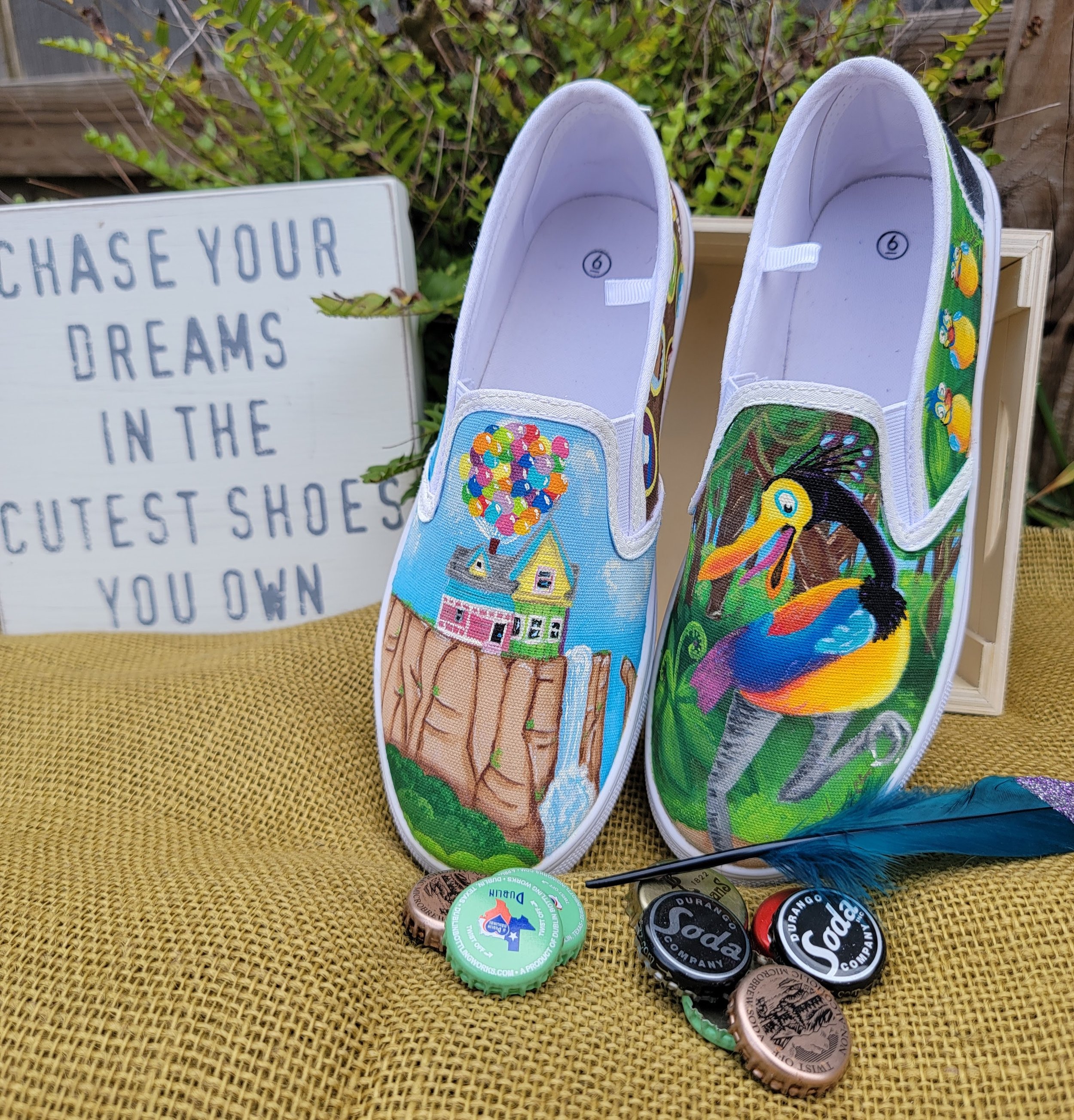In this detailed image, we see a pair of white, slip-on sneakers adorned with intricate, hand-painted designs, perfect for an Etsy product listing. The left shoe features a colorful cartoon-like bird with a vibrant body and a long black neck, looking down at the ground. Surrounding the bird are three smaller birds on the side panel, adding a whimsical touch. The right shoe showcases a scene reminiscent of the movie "Up," with a house suspended by numerous colorful balloons, appearing to float next to a cliff and waterfall backdrop. 

The shoes rest on a lumpy burlap sack-like material, creating a rustic setting. In front of the shoes, there are several bottle caps in various colors, including black, green, and gold, some with the word "soda" and others with different inscriptions. A blue feather lies directly in front of the shoes by the bottle caps, adding to the artistic display. To the left, a white painted sign with blue uppercase letters reads, "Chase your dreams in the cutest shoes you own." In the background, there is a small houseplant adding a touch of greenery to the scene. The inside of each shoe is visible, marked with the size "8."